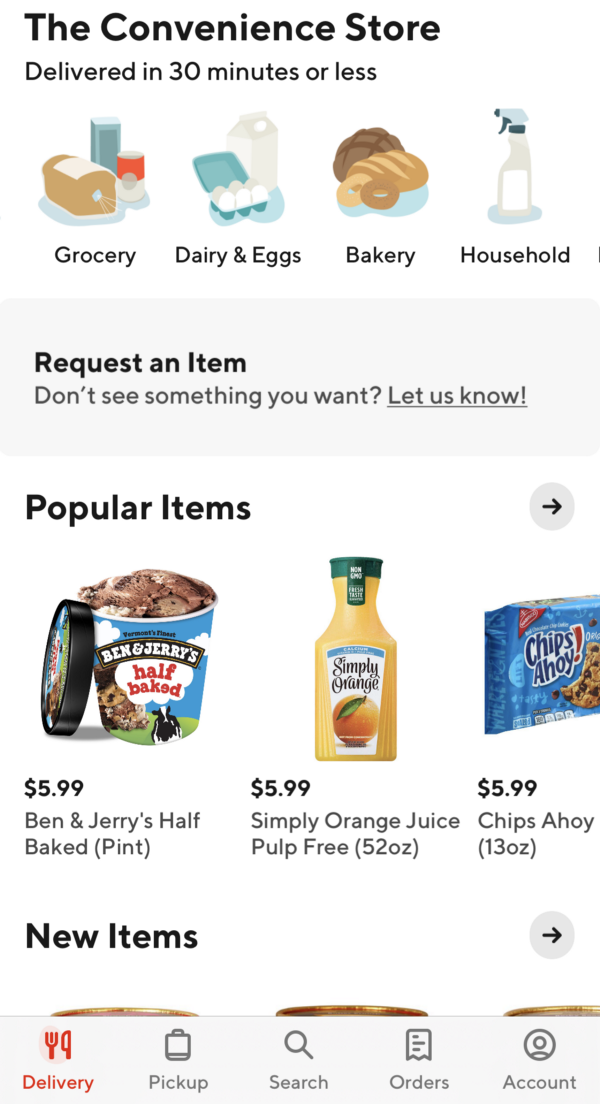**Detailed Caption:**

An advertisement for a convenience store's delivery service promises "The Convenience Store Delivered in 30 Minutes or Less" in bold black text prominently displayed at the top. Below this headline, an illustrative section showcases various grocery items: a loaf of bread, a can of soup, and a blue container. Adjacent to this section is another drawing under the "Dairy and Eggs" category, featuring a half-dozen white eggs in a blue carton and a carton of milk placed behind it.

The "Bakery" category is illustrated with a colorful donut and two freshly baked loaves of bread. The final category, "Household," includes a drawing of a spray bottle, indicating cleaning supplies. Beneath these categories, black text encourages customers to "Request an item. Don't see something you want, let us know."

Following this, the "Popular Items" section is introduced, displaying tempting product images with prices: Ben & Jerry's Half Baked ice cream with the lid off for $5.99, Simply Orange orange juice for $5.99, and a bag of Chips Ahoy cookies also for $5.99. At the bottom, the ad mentions a "New Items" category, suggesting fresh additions to their ever-expanding inventory.